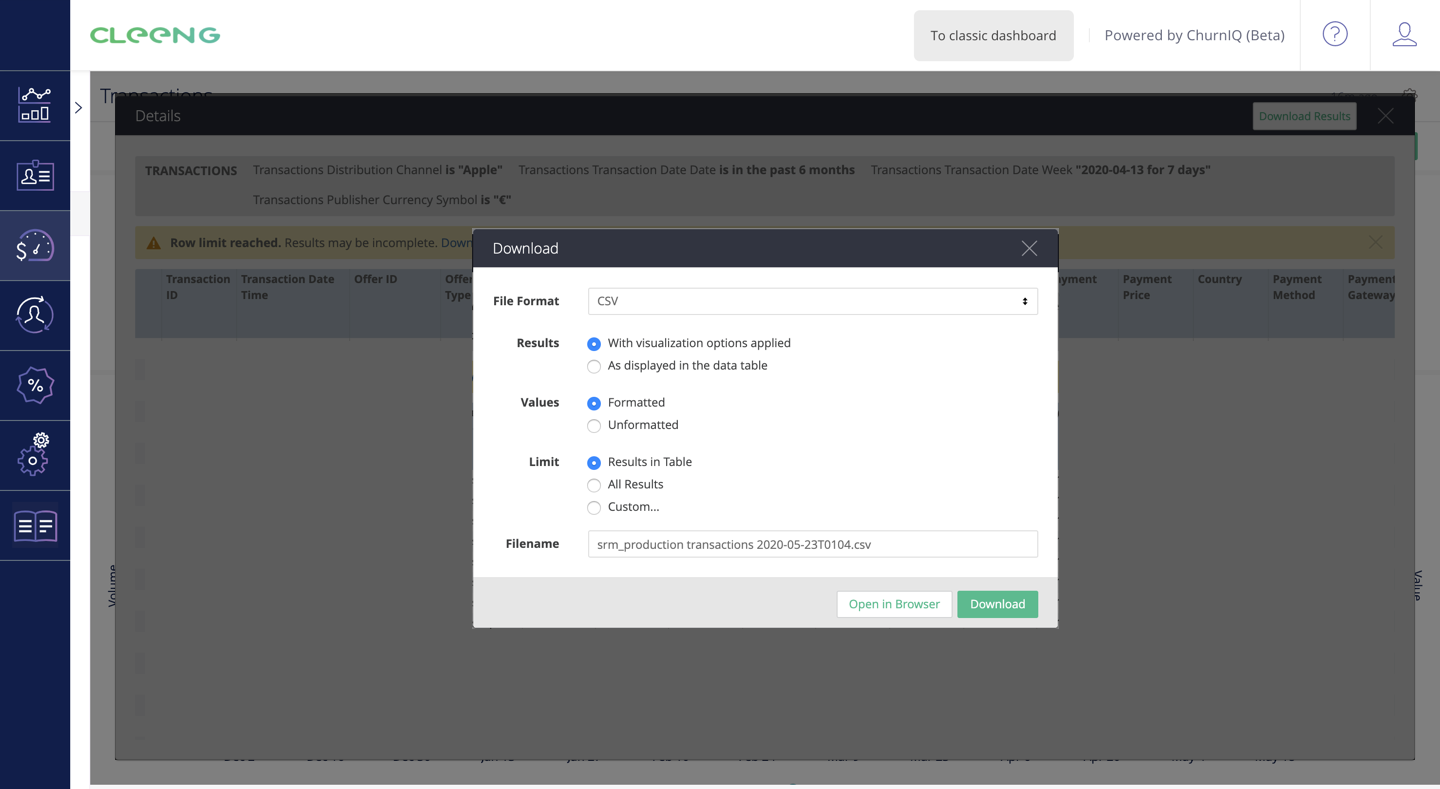The image is a detailed screenshot of a section of a website's user interface. At the top left corner, against a white background, the word "Cling" is displayed in green text. To its right, there is a gray button with black text that reads "To Classic Dashboard." Adjacent to this, there is another button, white with black text, that says "Powered by Churn IQ Beta."

Below this header section, there is a content area with a variety of interface elements. Dominating the top of this content area is a black banner displaying the word "Download" in white text, located at the upper left corner of the banner. Just below the banner, the left side of the screen features bold black text that reads "File Format." To the right of this text, there is a dropdown box that currently shows "CSV" as the selected option.

Underneath the file format section, the word "Result" appears in bold black text, followed by descriptions: to the right, "With Visualization Options Applied," and beneath this, "As Displayed in the Data Table."

At the bottom of the section, there is a bold text label "Values," accompanied by the label "Limit." At the bottom right corner, there is a white action button labeled "Open in Browser." The overall background of the web interface is grayed out, making the white content box and black banner stand out clearly.